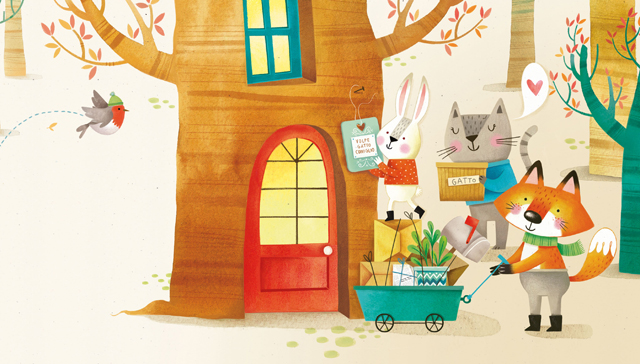In this detailed illustration reminiscent of a children’s book, set against a tan, forest-like background with a textured, almost paper-like cutout feel, we see a whimsical scene featuring charming cartoon animals. At the center, there's a large tree with realistic wood grain patterns, adorned with a red door with an oval archway, from which yellow light emanates, and a blue-framed window above it. The focal point includes a fox with a green scarf, light gray pants, and black boots pulling a wagon full of packages and a potted plant towards the tree. Beside the fox, a gray cat dressed in a light blue sweater, characterized by whiskers and a tail, carries a box labeled "Gato" with a speech bubble containing a pink heart. Completing the group, a rabbit dressed in a red sweater with yellow dots hangs a sign outside the doorway. Off to the left, a red, white, and gray bird wearing a winter hat is mid-flight, adding to the lively, bustling atmosphere of this enchanting forest scene.